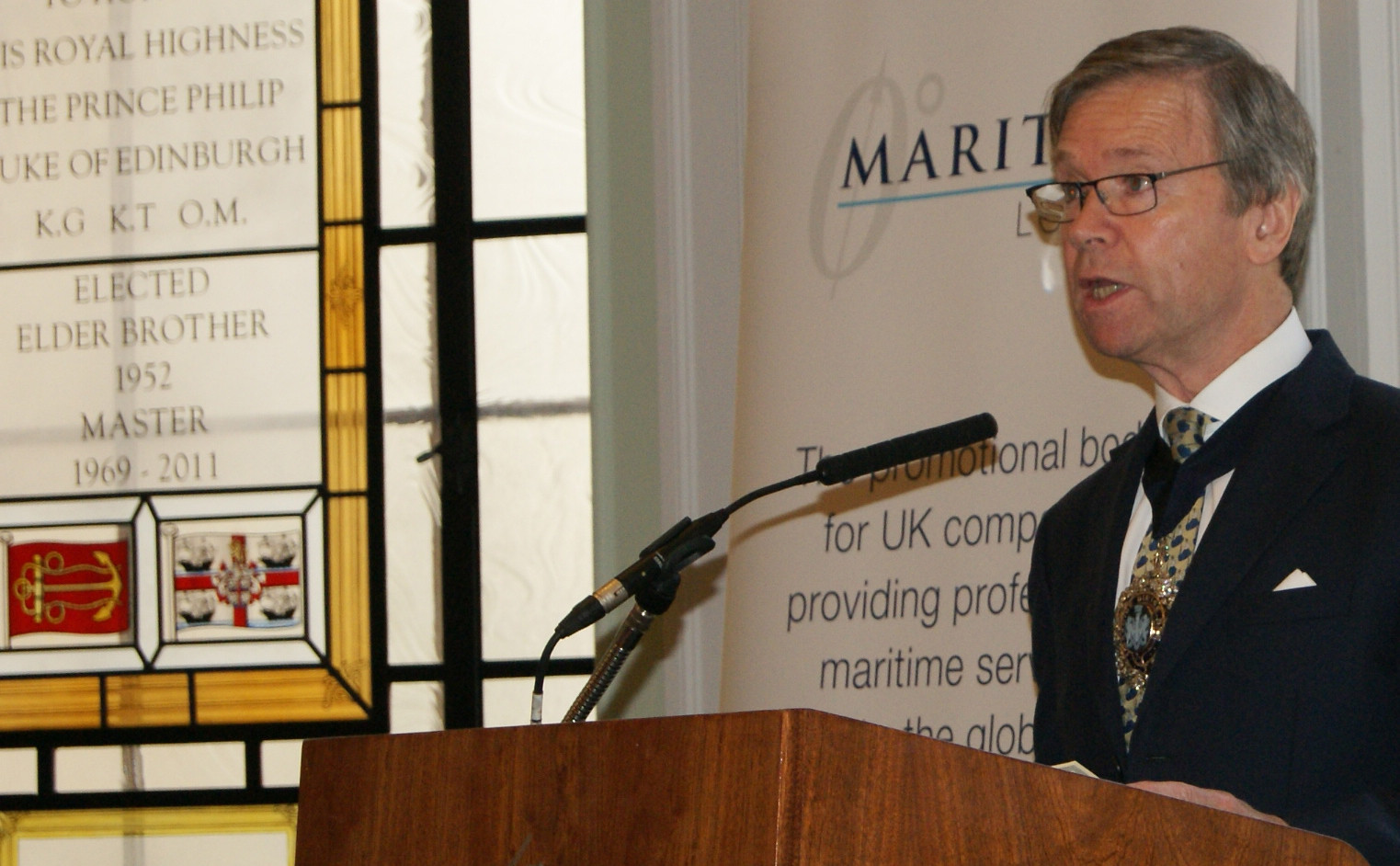A detailed photograph captures an indoor setting where an older man, with short, graying hair, stands at a wooden podium equipped with a black microphone. The man, seen from the waist up, is dressed in a black sports jacket over a white shirt, and sports a printed tie with beige and blue dots. A gold medallion with a light blue center hangs over his tie. He also wears glasses with black frames. Behind him, partially obscured by his head, is a white sign, with visible letters spelling "MARIT," hinting at maritime promotional services in the UK. To the left, a stained glass window panel references "His Royal Highness, the Prince Philip, Duke of Edinburgh, Elected Elder Brother 1952, Master 1969-2011," with images of flags displayed below.